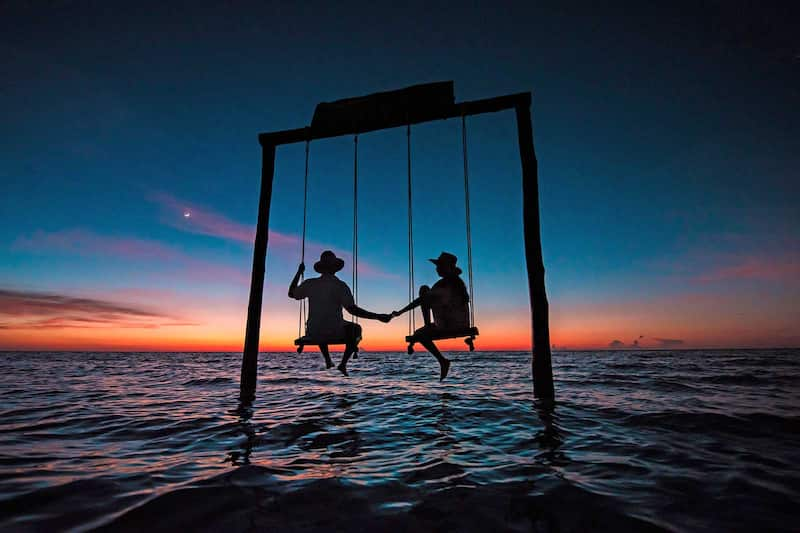The photograph captures a serene image of a swing set partially submerged in a body of water, possibly the sea or ocean, during an orange-tinted sunset. The swing set is constructed from tall, skinny wooden poles, approximately 10 to 12 feet high, with a horizontal beam connecting them at the top. Attached to this beam are two separate swings. Seated on the swing to the left is a person wearing a cowboy hat, holding hands with another person facing them on the right swing, who is also wearing a sun hat. The late evening sky above is a gradient of dark blue transitioning to the vivid oranges, reds, and yellows of the setting sun. The water below is a deep blue with slight ripples, giving the scene a tranquil yet slightly dynamic feel. An almost imperceptible moon can be seen in the darkening sky. Small clouds linger to the left, adding to the ethereal beauty of this romantic and picturesque setting.